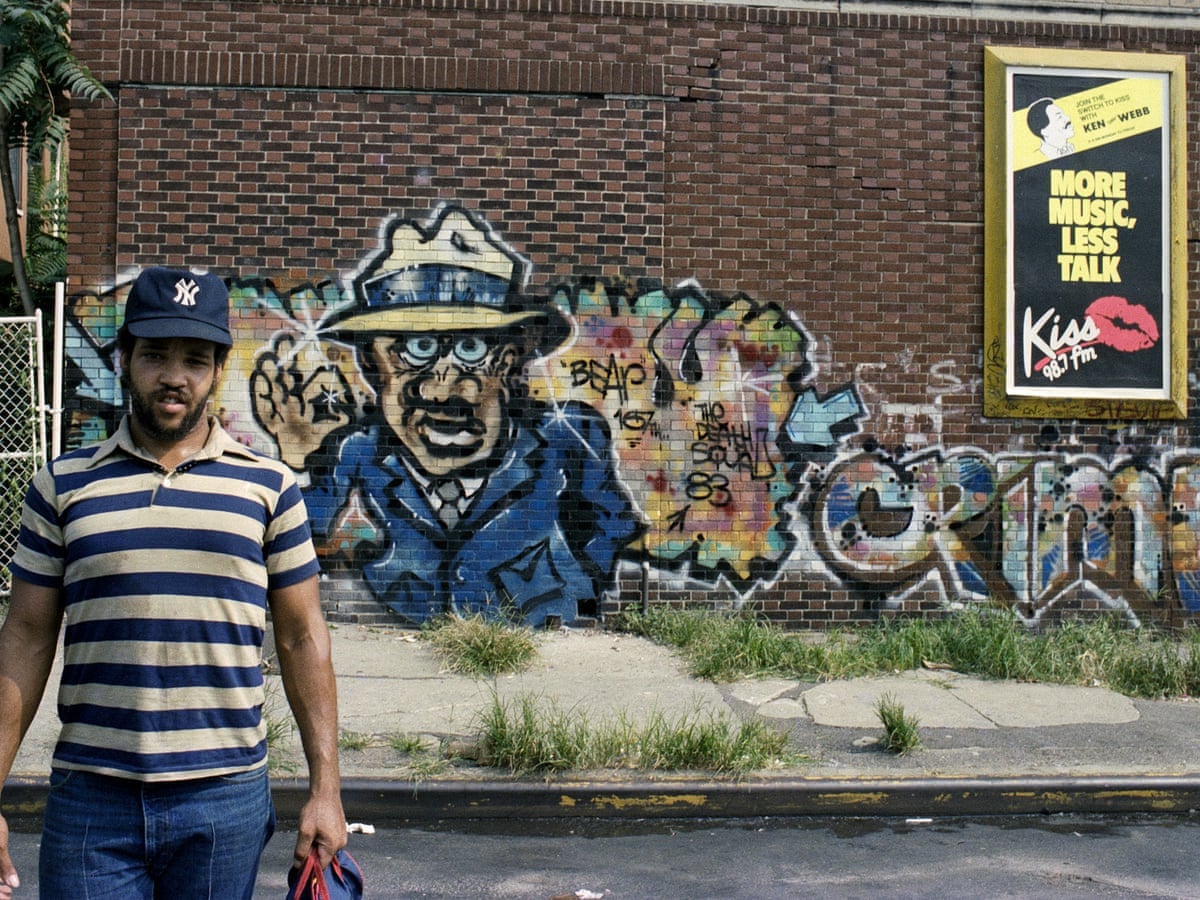In this photograph, a young Black man with black hair and a beard poses confidently in front of a vibrant graffiti mural. He's sporting a dark blue Yankees cap, featuring the iconic white "NY" logo, a tan and blue striped collared shirt with three buttons, and denim jeans. Slung over his shoulder is an athletic bag, hinting that he may be the artist behind the mural.

The mural itself showcases a cartoonish figure of a Black man dressed in a blue suit, blue bowtie, and a tan hat, making an A-OK finger gesture. The background is adorned with additional graffiti elements and a retro, slightly dated feel. To the right of the man, a vintage poster stands out, proclaiming "More Music, Less Talk, Kiss 98.7 FM," complete with a kiss mark, hearkening back to an era when this radio station was prominent in New York.

The combination of the man's attire, the mural, and the vintage poster suggests that this photograph captures a slice of old New York, likely from the 1980s, providing a glimpse into a vibrant and artistic moment in time.